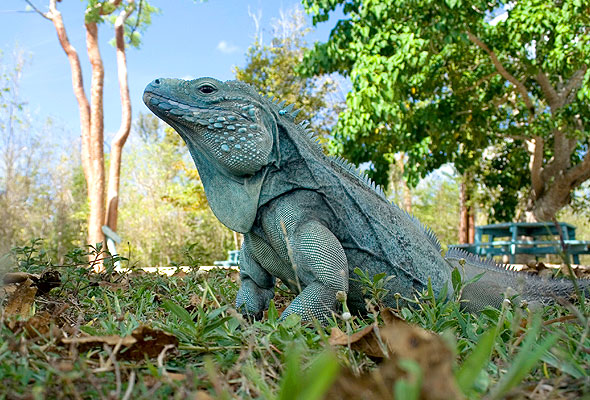The photograph captures a dynamic scene from ground level, providing an intimate close-up view of a striking lizard positioned at the very center of a wide vertical rectangular frame. It is daylight, evident from the vibrant blue sky that spans the background. Dominated by various shades of green, the surroundings feature trees and shrubbery, contributing to the natural ambiance. 

To the right, a blue picnic table is partially visible against the verdant setting. At ground level, numerous green blades of grass interspersed with brown leaves frame the lower part of the image, emphasizing the earthy environment. 

The lizard, specifically an iguana, stands as the central subject, showcasing a unique blend of light blue and teal hues, reminiscent of tarnished copper, akin to the Statue of Liberty's patina. This iguana exhibits a proud posture: its front legs are elevated, pushing up its chest with the head turned slightly up to the left, and its tail trailing behind. Its mouth remains closed, and it gazes upward with dark, scaly eyes. 

Noteworthy is the ridge along its spine, composed of small, raised spines or skin parts that resemble delicate blades. The textures and colors of its tough, scaly body are clearly defined, providing a vivid display of its physical characteristics. 

This photograph expertly balances the majesty of the lizard and the serene, daylight backdrop, capturing a moment in nature that feels both tranquil and vibrant.